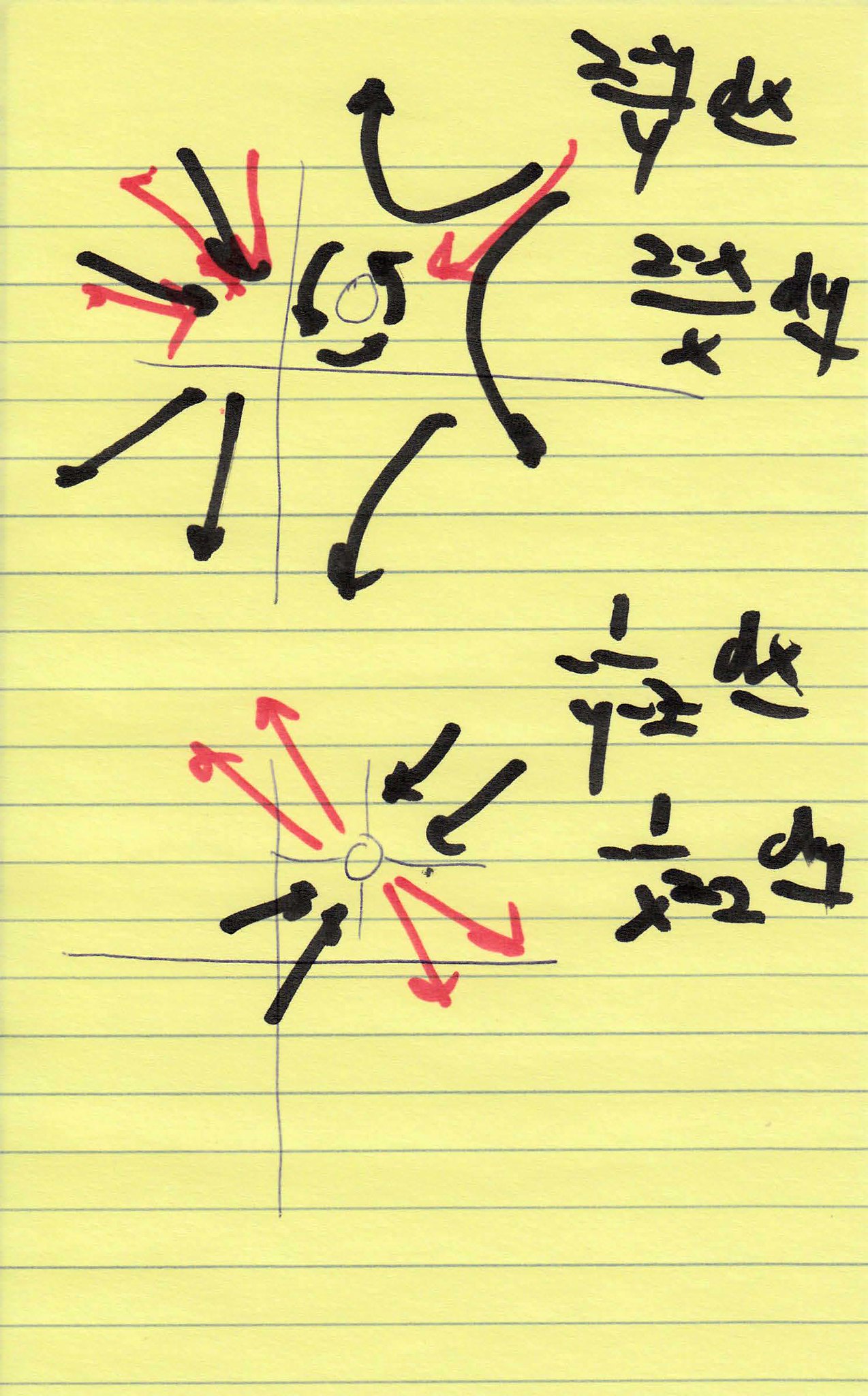The image features a yellow piece of paper with blue lines. At the top, there is an equation that reads "2y/y dx," which is underlined. Below this, the equation continues with "2 - x" followed by a line that separates it from "x dy." It further includes "1 1/2 dx" and "1/32 dy."

The paper also contains multiple arrows in black and red. Specifically, there's a black arrow pointing upward, followed by a series of alternating red and black arrows pointing downward. There is one red arrow pointing upward, and then three more black arrows pointing downward. The second set of arrows has four red arrows—two pointing upward, and two pointing downward—as well as two black arrows pointing upward and two more black arrows going sideways.

The rest of the page is blank, emphasizing the mathematical expressions and the various directions of the arrows, all depicted in red and black ink, on the yellow lined paper.